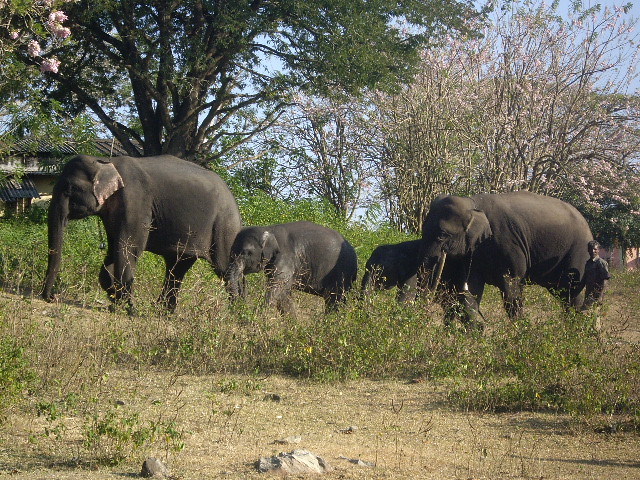In this photograph, a small group of elephants is depicted walking through a natural landscape. Dominating the scene in the middle is a large, dark gray elephant with distinctive pink stripes at the tips of its ears, flanked by another large elephant on the right side. Two younger elephants, considerably smaller yet walking in between the two adults, make up the center of the line. The ground they traverse features sparse grass, weeds, and sporadic rocks, while the background reveals a mix of trees—including some dead, brown, and spindly ones without leaves and a couple of more robust trees. One of these trees is particularly notable for its large green branches reaching skyward and another for its pale pink blossoms. 

A man, who appears to be herding the elephants, stands next to the adult elephant on the right. He has black hair, olive skin, and is wearing a dark grayish-green, short-sleeved shirt. The man appears to be holding a tool, adding a dynamic element to the otherwise serene yet slightly rugged natural setting.